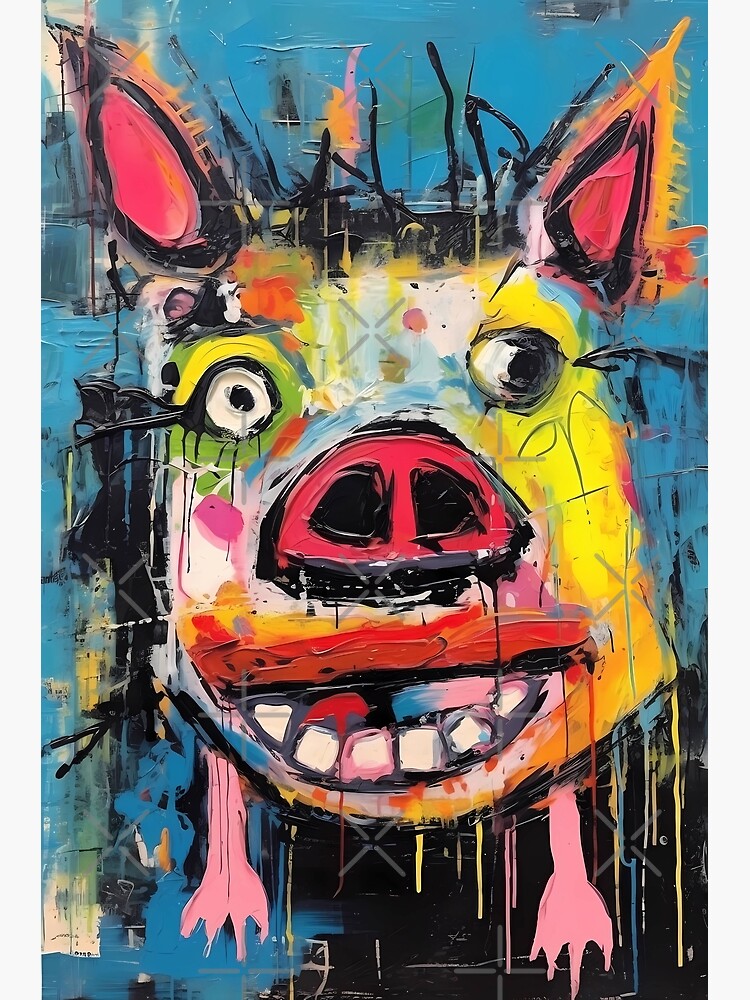This abstract painting depicts a whimsical pig face against a primarily blue and black background. The pig's face is vibrantly colorful, featuring a red or reddish-pink snout, yellow and white patches, and googly eyes that are different sizes. The pig has pink ears outlined in black and a wide, grinning mouth displaying large white teeth bordered by various colors like pink, blue, red, and neon green. The expressive face also has streaks of paint dribbling down, adding to the chaotic charm of the piece. Draping from the bottom of the face are two human-like pink arms with four fingers each. Additionally, there are grey crosses scattered across the image, and accents of orange and white add to the painting's dynamic and messy feel.